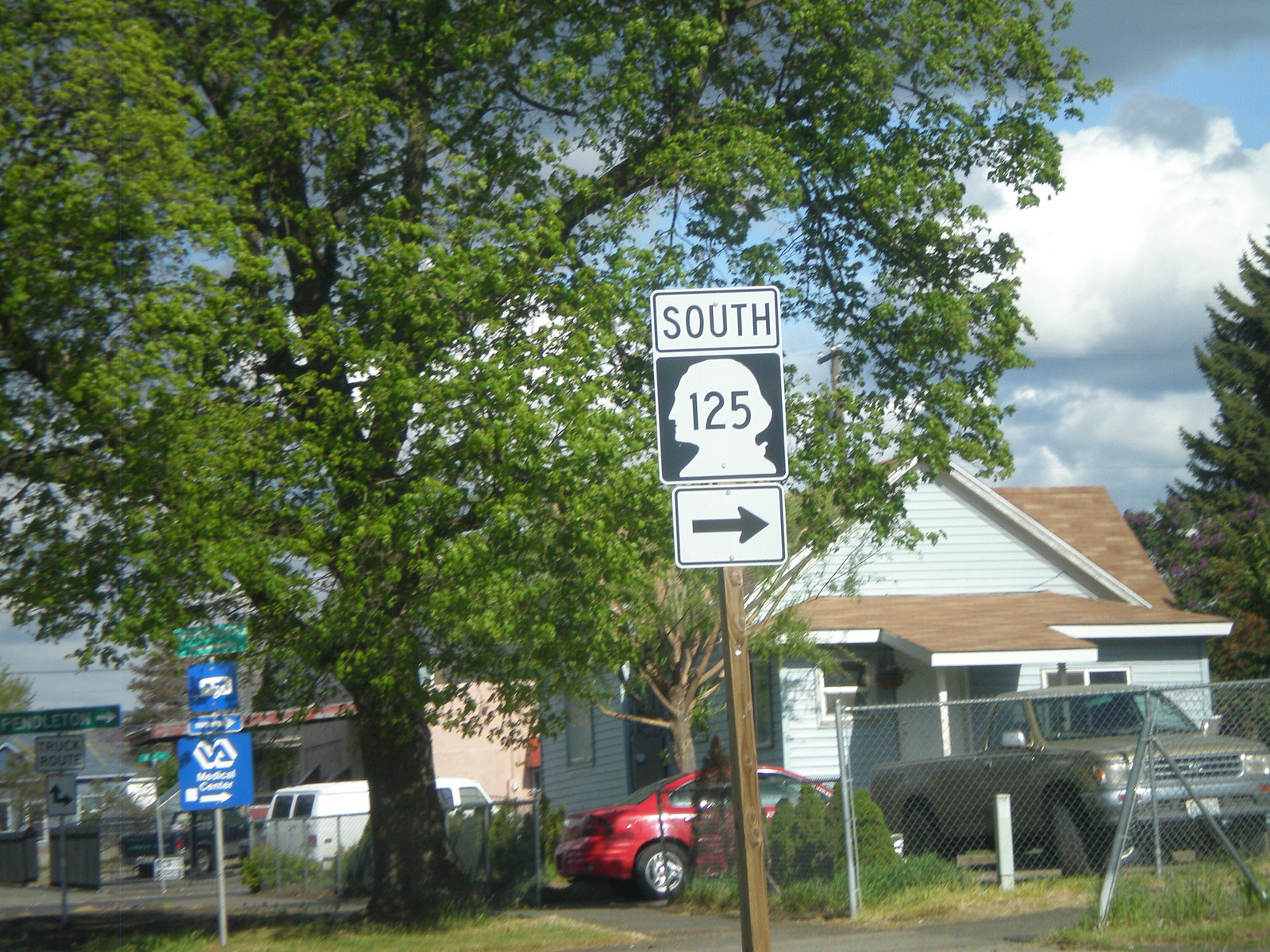The image depicts a quaint residential neighborhood featuring a small, possibly light blue or green, bungalow-style house. Positioned prominently beside the house is a large tree with lush green leaves and dark brown bark. In front of the house, a red compact car and a brown pickup truck are parked behind a chain-link fence.

A white traffic sign with a black outline of a historical figure, possibly a colonial man's head, displays the number "125" and the word "South" above it. Below the number, an arrow points to the right, indicating the direction of South Highway 125. Nearby, there is also a blue sign with a bus icon, suggesting a bus stop, and another sign indicating directions to a medical center.

In the background, behind the tree and the house, a white van and a dark-colored pickup truck can be seen. The backdrop also includes what appears to be a small grocery store or perhaps a gas station with an overhang. This sign-rich scene suggests a well-traversed route with multiple transportation options and a touch of historical flair.